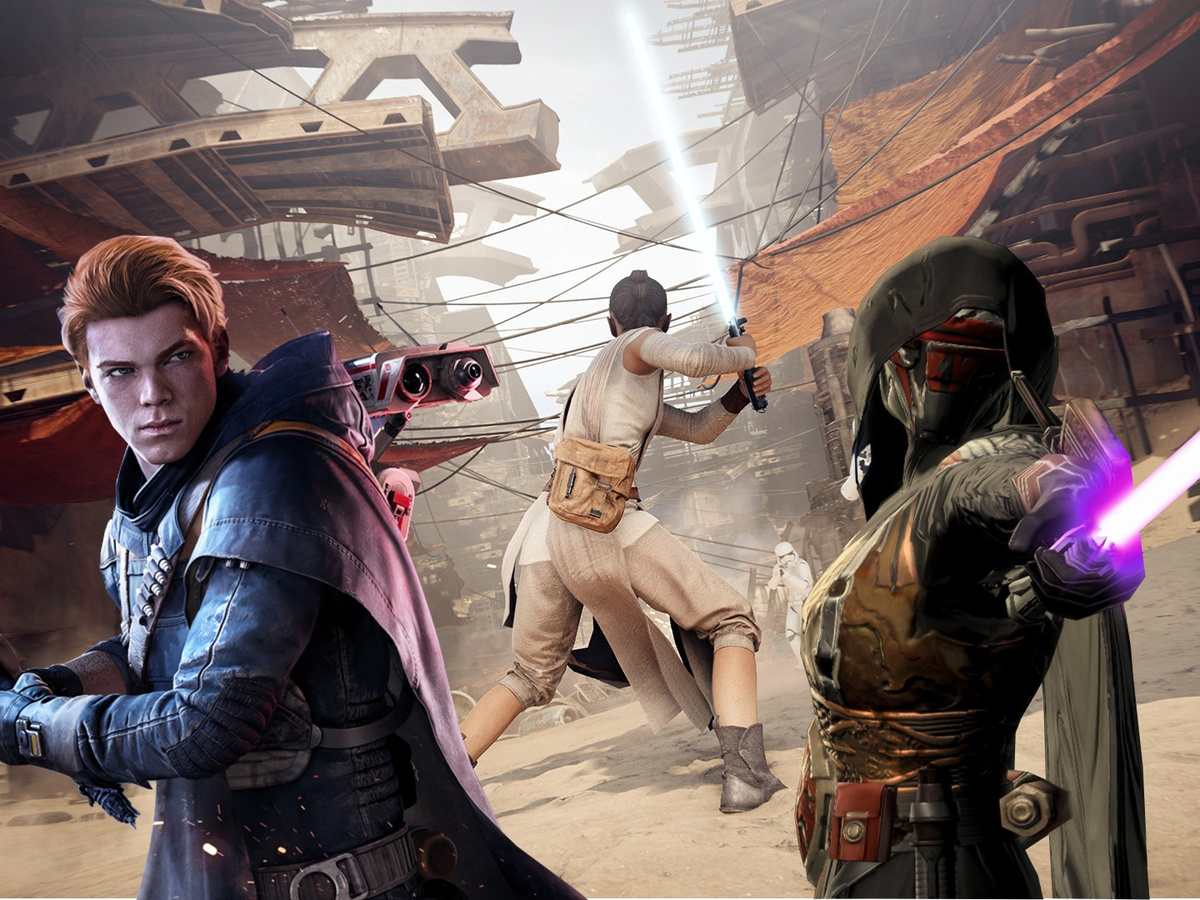The image is a highly detailed computer-generated art piece set in the Star Wars universe, likely depicting a scene from the newer movies. The central character, identified as Rey, stands with her back to the viewer, poised and gripping a white lightsaber. She is dressed in beige attire with a matching bag slung over her shoulder. The setting is a desolate, sandy landscape, possibly the city of Tatooine, featuring derelict buildings adorned with orange tapestries and crisscrossing wires.

To the left of Rey is a determined-looking young man with reddish-orange hair, dressed in a distinctive blue uniform and cape. A bandolier with bullets is strapped across his chest. He is accompanied by a robot peeking from behind him, both gazing towards the right.

On the right side stands a mysterious figure garbed in a dark yellowish-brown metallic uniform, cowl, and mask. This figure wields a striking purple lightsaber and emanates an ominous presence, suggesting an alignment with the dark side or possibly a Sith Lord. The detailed background of the scene, draped in the Star Wars aesthetic, further enriches the narrative depicted by these iconic characters.